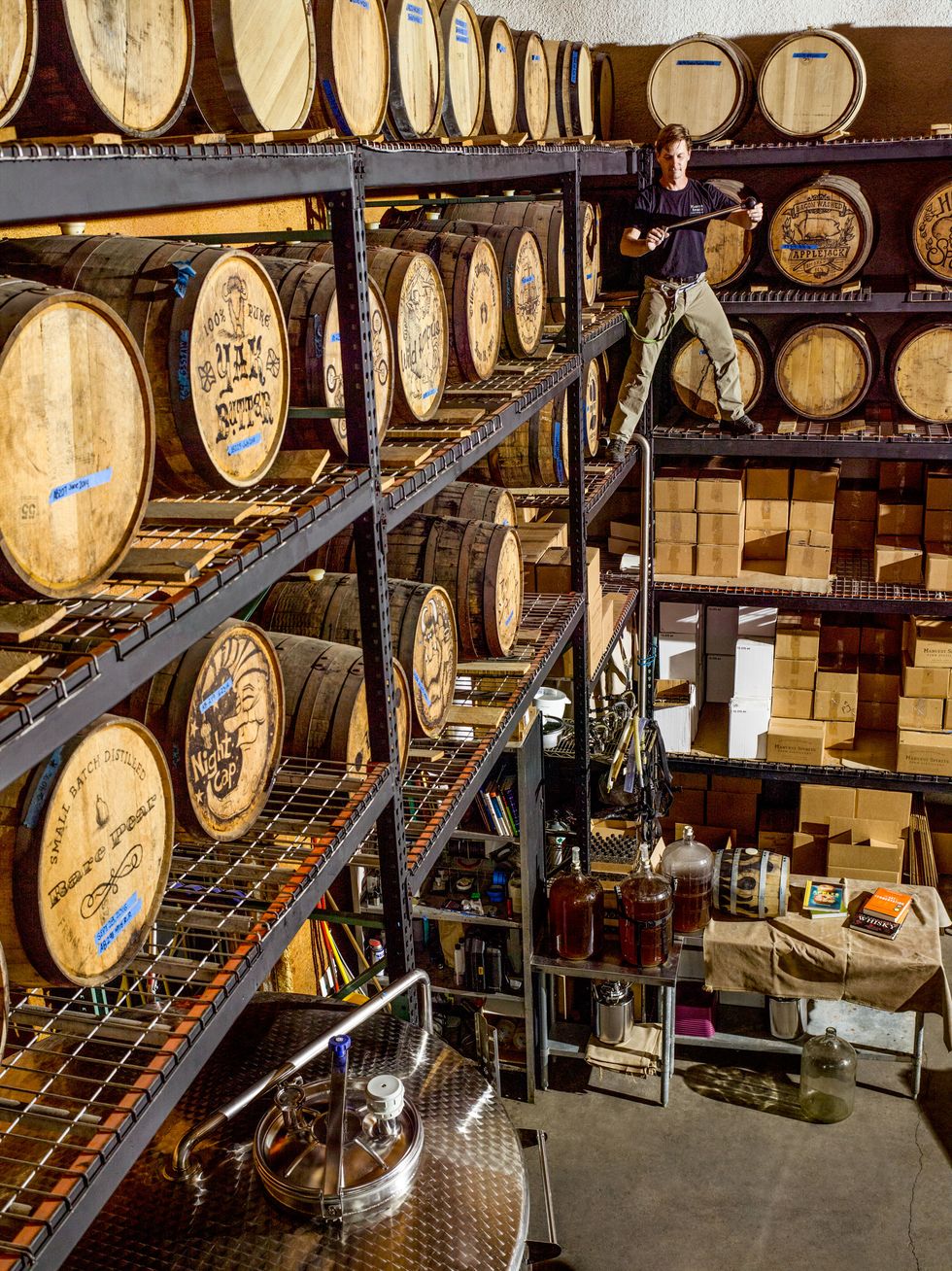The photograph captures the interior of a large warehouse or brewery with towering shelves reaching up to a very tall ceiling, estimated around 30 feet. The shelves are laden with wooden barrels, displayed sideways, likely used for storing beer, whiskey, or wine. In the background, where two shelving units meet, a man is perched high up near the top shelves. He is wearing a dark-colored shirt—either purple or dark blue—and khaki pants. The man, who appears to have reddish-brown or dirty blonde hair, is secured with a safety harness and is seen balancing with one foot on each side of the shelving, holding an object that might be a ruler. Below him, the concrete floor shows a noticeable crack and supports additional items: a table with large 10-gallon jars filled with a brown liquid, and various square cardboard boxes, tan and white, neatly arranged on the lower shelves. Additional kegs and boxes fill the area, emphasizing the storage purpose of this expansive space.